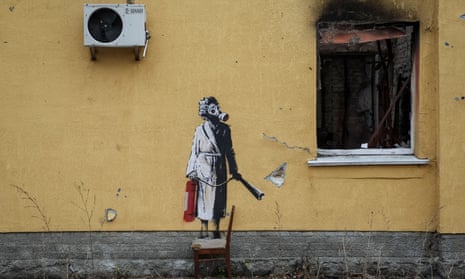This color photograph captures the outside of an aged, yellow building, likely in a slum or possibly damaged by fire. The wall, which rests on a concrete foundation, features a stylized, Banksy-like drawing. In the graffiti, a person in curlers and a long, white bathrobe—blackened by smoke—is depicted standing on a brown wooden chair. This figure wears a gas mask and holds a red fire extinguisher, aiming the nozzle towards an open window with a white windowsill. The window appears shattered and charred, with soot and extensive smoke damage indicating that the interior has been gutted by fire. Mounted on the upper left section of the wall is a white air conditioning unit with a black fan. The entire scene evokes a sense of decay and tragedy, inviting empathy for the former inhabitants while showcasing the poignant street art.